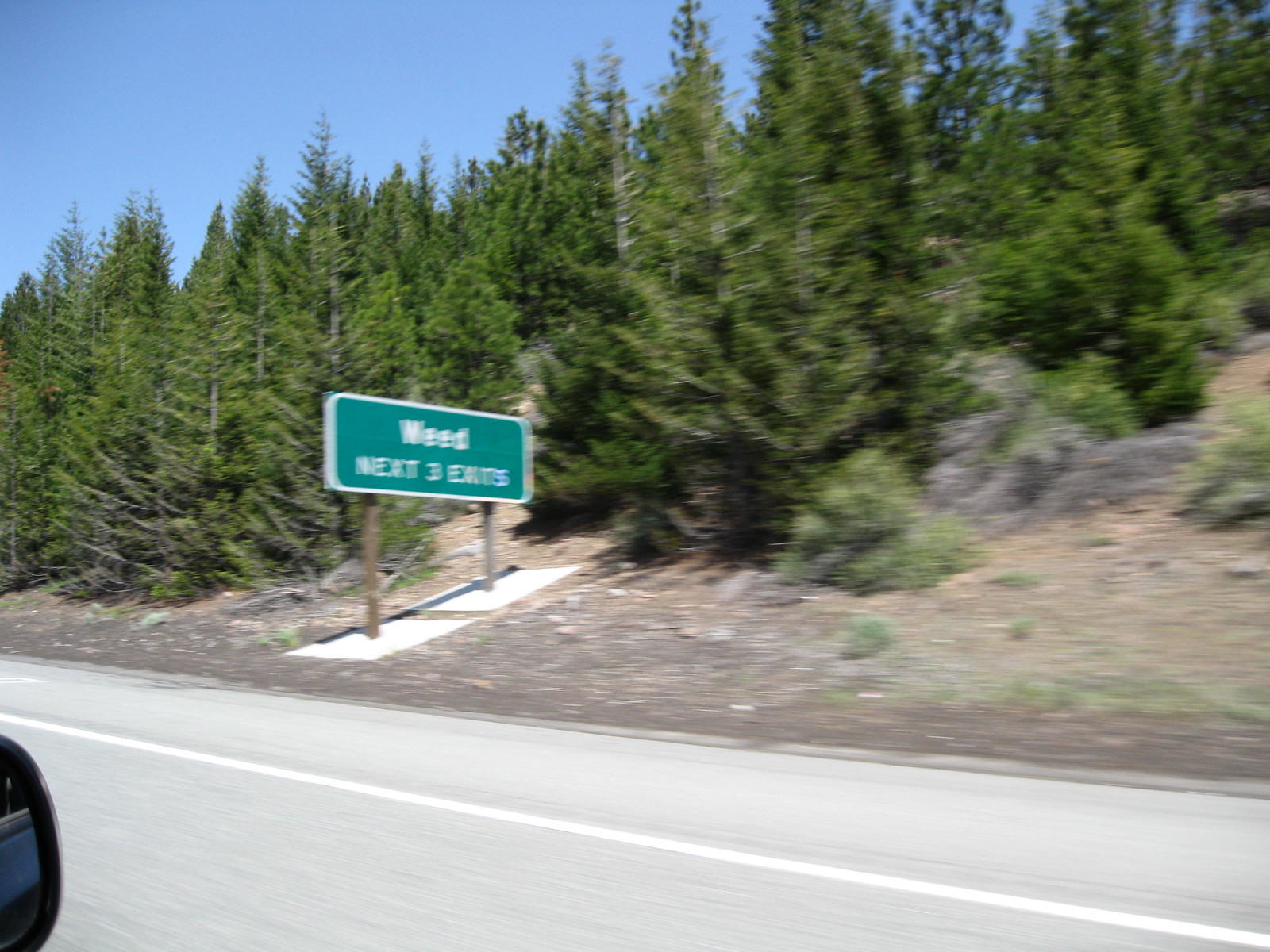The image captures a blurred view from the passenger side of a moving vehicle on a highway. In the bottom left corner, the faint outline of the car's side mirror is visible, indicating the photo is taken from inside the car. To the right, the highway becomes clear, showing the right-hand lane bordered by a white line. Beyond the lane, there's a grassy shoulder leading up a dirt embankment dotted with medium-sized pine trees. Prominently in the center-left of the photo, there's an elongated green road sign with white letters stating "WEED, next three exits." This contributes to a distinctly American roadside scenery. The upper portion of the image gives off a sense of motion, adding to the slightly blurred effect as the car travels down the highway.